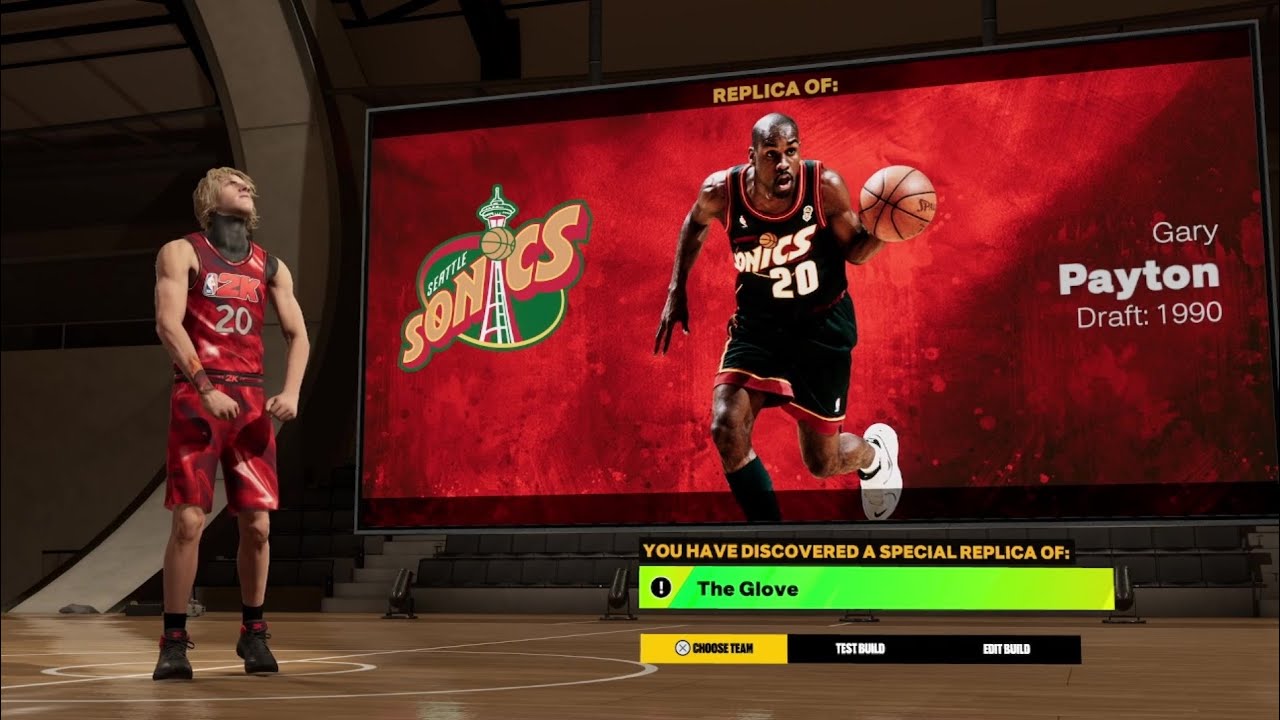This screenshot from a video game features a large monitor situated in the upper right section of the screen. The monitor is outlined in gray with a black banner at the top that reads "Replica of." Below the banner, the image showcases an African-American man dressed in a black basketball uniform with red and orange piping. The uniform, emblazoned with the number 20 and the name "Sonics," represents the Seattle SuperSonics. The player, who is gripping a basketball in his left hand, is mid-motion with his left leg raised, showcasing his white and black sneaker.

To the left of the player, there is a vibrant logo that reads "Seattle Sonics" in green, orange, white, and red. Below the image of the player, the text "You have discovered a special replica of" appears, followed by "The Glove" in a green box. Located beneath this text are the option buttons labeled "Choose Team," "Test Build," and "Edit Build."

In the upper right corner above the player, additional text provides context: "Gary Payton" and "Draft 1990," indicating the player’s name and draft year.